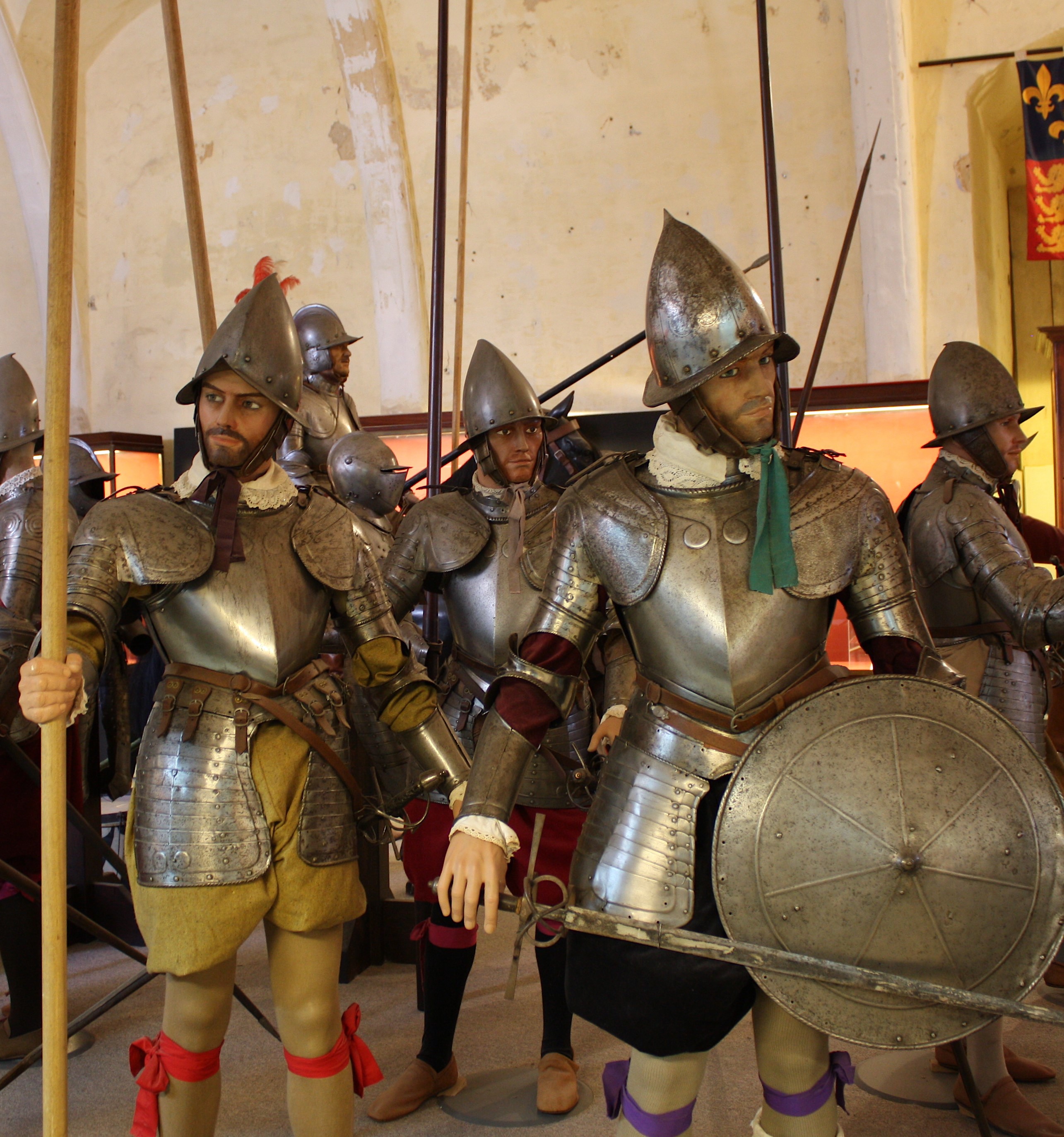The image depicts a collection of highly lifelike wax figures, meticulously crafted to resemble medieval warriors. Each figure is adorned in partial suits of authentic-looking armor, including breastplates and pointed helmets, known as sallets. These figures lack greaves, with their lower bodies instead covered by poofy shorts and shirts visible from beneath the armor. The foreground features two prominent figures: the one on the left wears black poofy shorts paired with a red shirt, and the one on the right dons a pale green shirt and matching poofy pants. Both figures are equipped with different weaponry; the left figure holds a long sword and a shield, while the right figure grips a pike.

Behind these figures, more similarly dressed and armored wax statues are arranged, standing on a brown floor and enveloped by a canvas enclosure. Notably, one figure on the left side, slightly behind the front one, wears beige shorts with red ribbons around the knees, holding a vertical stick-like weapon. The background is equipped with natural lighting, enhancing the clear visibility of the intricate details. A black, red, and gold banner is visible in the top right corner against a white wall, suggesting a medieval-themed setting. The overall scene is vivid and bright, capturing the viewer's attention with its realism and historical accuracy.